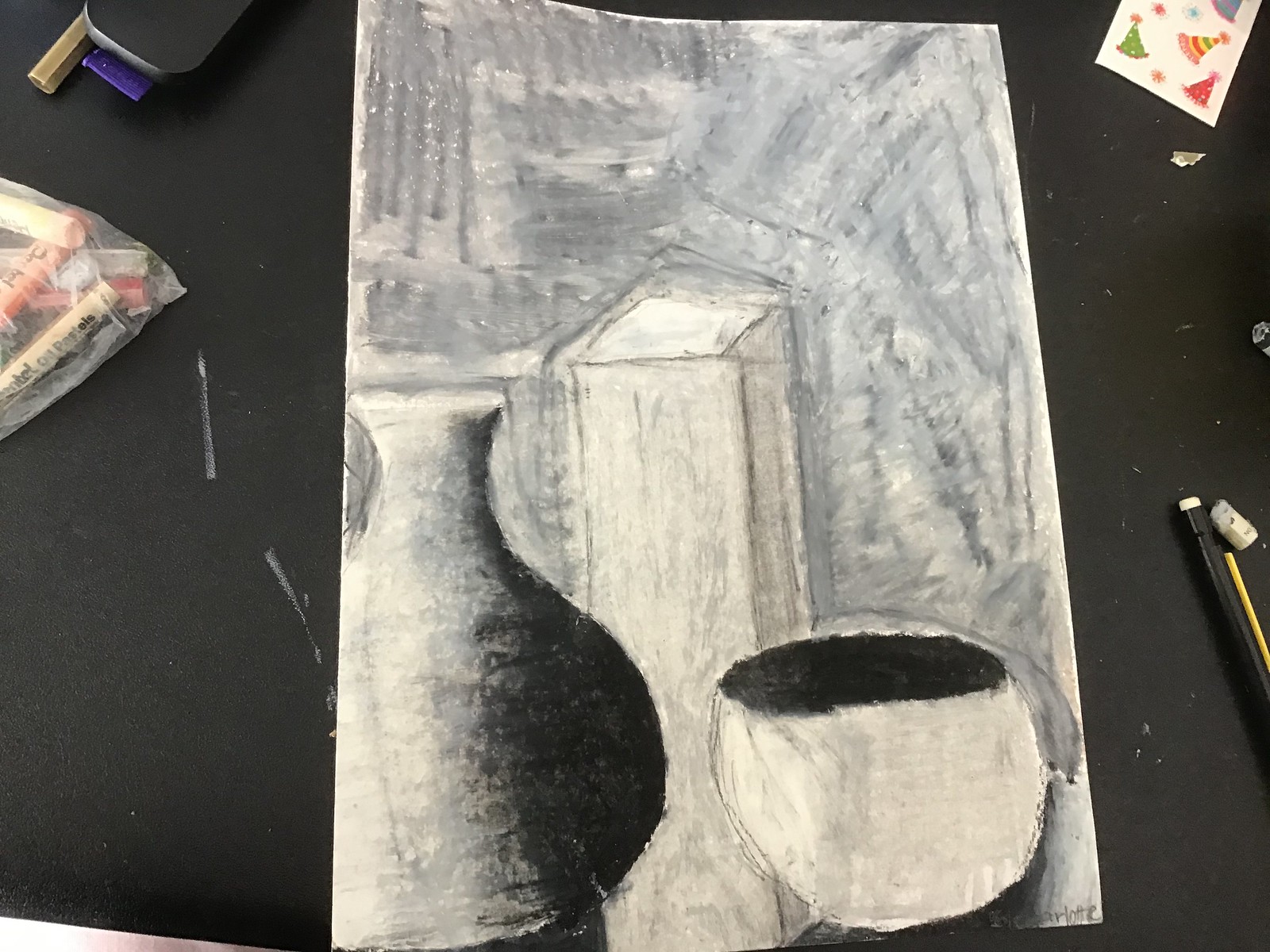In this image, we see an artistic composition viewed from above, centered on a black art easel or table. The focal point is a large piece of paper featuring an intricate pencil sketch that reveals the artist's attention to detail and significant investment of time and thought. The scene within the sketch captures a variety of objects with meticulous shading that ranges from deep blacks to stark whites, adding depth and realism.

On the lower left side of the drawing, there is a vase with a narrow top and a broad base, expertly rendered to showcase its dimensionality through intense shadowing. Beside the vase, a small white bowl is depicted with a completely blackened interior, contrasting sharply against the more textured elements around it.

In the background of the sketch, subtle details suggest the presence of furniture or architectural elements. A vertical object, possibly the corner of a shelf, stands prominently, while the adjacent areas are filled with varying shades of gray, which could represent other pieces of wood or furnishings. The background transitions through light and dark patches, creating a dynamic and textured environment that fills the entire space.

In the lower right corner of the paper, the artist has signed their work with the name "Charlotte" in pencil, adding a personal touch to the piece. Surrounding the paper on the easel are several art tools and materials: pencils and what appears to be an eraser on the right side, and a small plastic bag positioned in the upper left corner.

This detailed setup not only highlights the artist's skill but also provides a glimpse into the creative process and the environment in which the artwork was created.